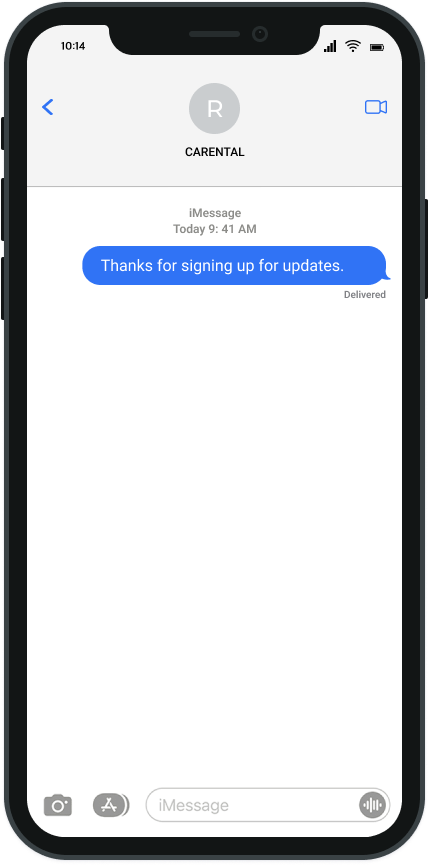The image portrays a screenshot of a cell phone's interface. The cell phone appears to be black, with clearly visible power and volume buttons—three on the left side and one on the right. The screenshot captures a page with a gradient background transitioning from light gray at the top to white at the bottom.

At the top of the screen, the time is displayed as 10:14 in black print. Directly below this, there is a black status bar featuring various icons: a partially filled battery icon indicating less than full charge, a Wi-Fi signal icon, and cellular signal bars.

Moving down to the central part of the screen, there is a prominent gray circle with a white, capitalized "R" inside it. Below this emblem, the text "Care Rental" is visible. An arrow pointing to the left and a video icon on the right side further accentuate this section.

Below this central area, a section dedicated to messaging is visible. It reads "iMessage Today 9:41 AM" followed by the message, "Thanks for signing up for updates," with the status "Delivered" indicated beneath the text.